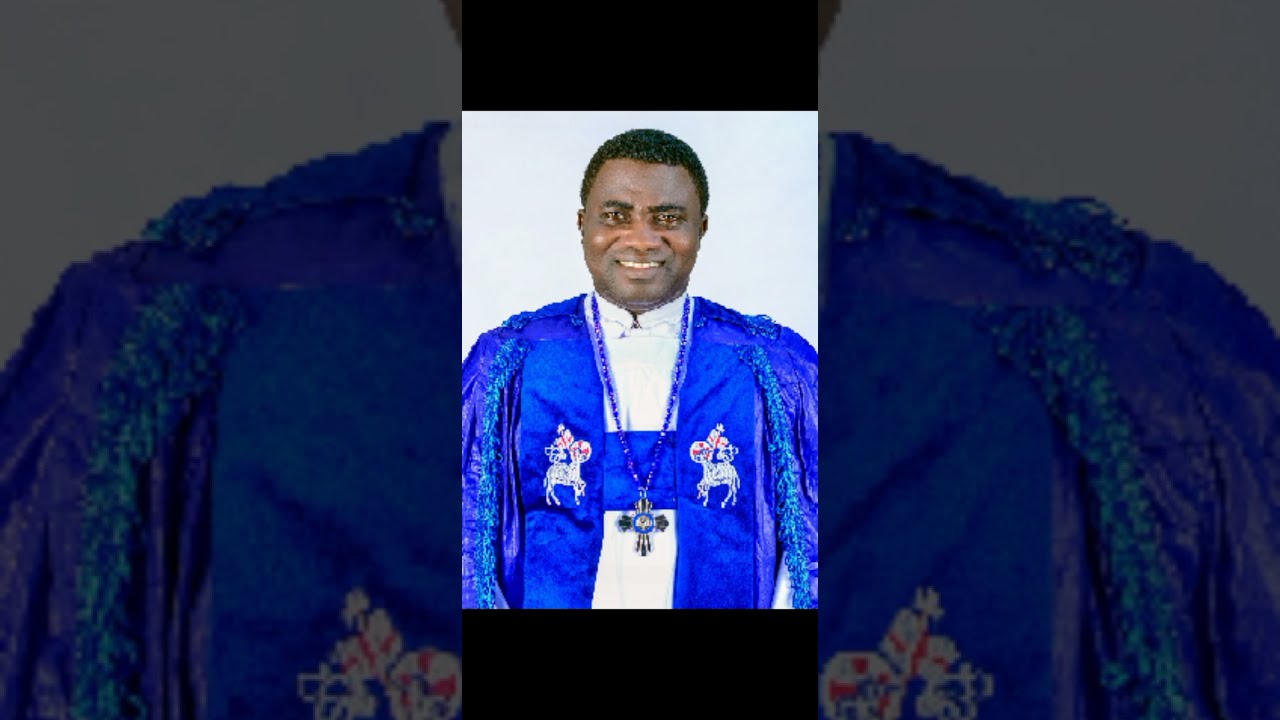The image features a dark-skinned priest with short curly black hair and thick eyebrows, slightly smiling and looking directly at the camera. He is dressed in a bright royal blue, shiny robe adorned with blue decorations on each sleeve. On both sides of his chest, there are white cavalier horse logos, possibly depicting knights riding on horseback, facing each other. The priest is also wearing a long, matching blue beaded necklace with a silver cross featuring a blue circular emblem in the middle, which hangs down to his stomach. Underneath the robe, he wears a white shirt with a notable blue stripe running down the center. The background of the image is a light, whitish-blue color.